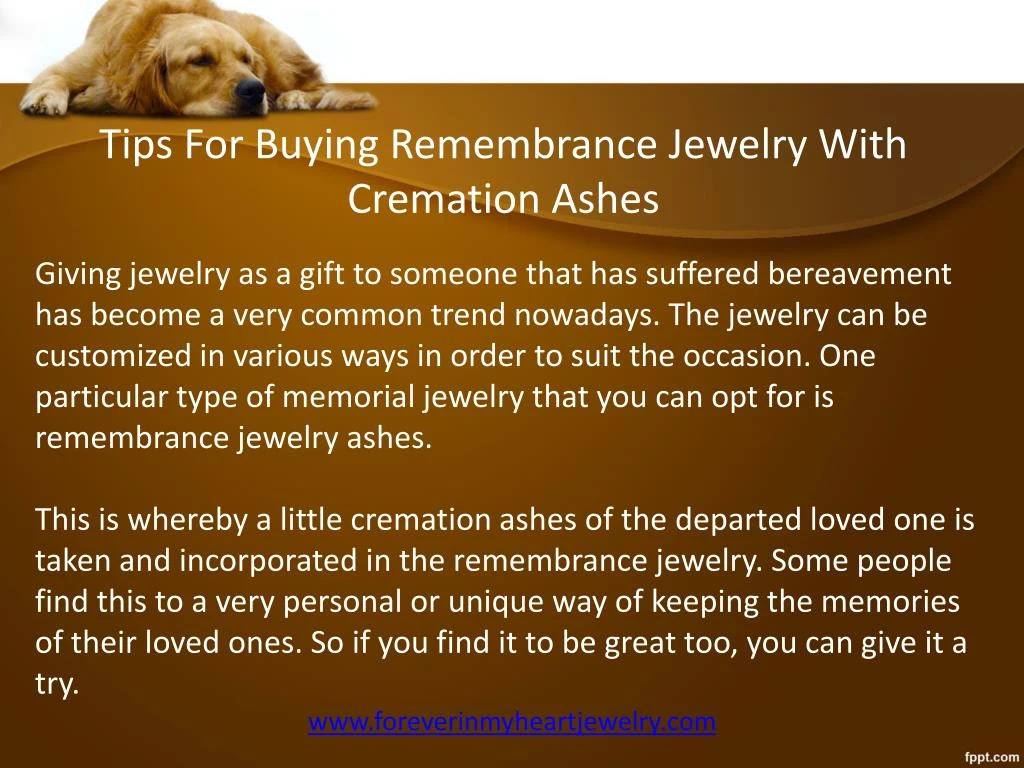The image is an advertisement for purchasing remembrance jewelry that incorporates cremation ashes. Set against a warm brown background, it features a somber golden retriever lying down in the top left-hand corner. The headline at the top reads, "Tips for Buying Remembrance Jewelry with Cremation Ashes," in white text. Below the headline, the ad explains that gifting jewelry to someone who has experienced bereavement has become a widespread trend. It mentions that this jewelry can be customized in various ways, highlighting a specific type known as Remembrance Jewelry Ashes, which incorporates a small amount of a departed loved one's cremation ashes. This type of jewelry is presented as a unique and personal way to keep the memory of loved ones close. The text encourages those interested to consider this option. At the bottom of the ad, there's a link to the website www.foreverinmyheartjewelry.com, although the specifics of the link are hard to read due to its blue text. Additionally, "fppt.com" is noted in the bottom right corner.